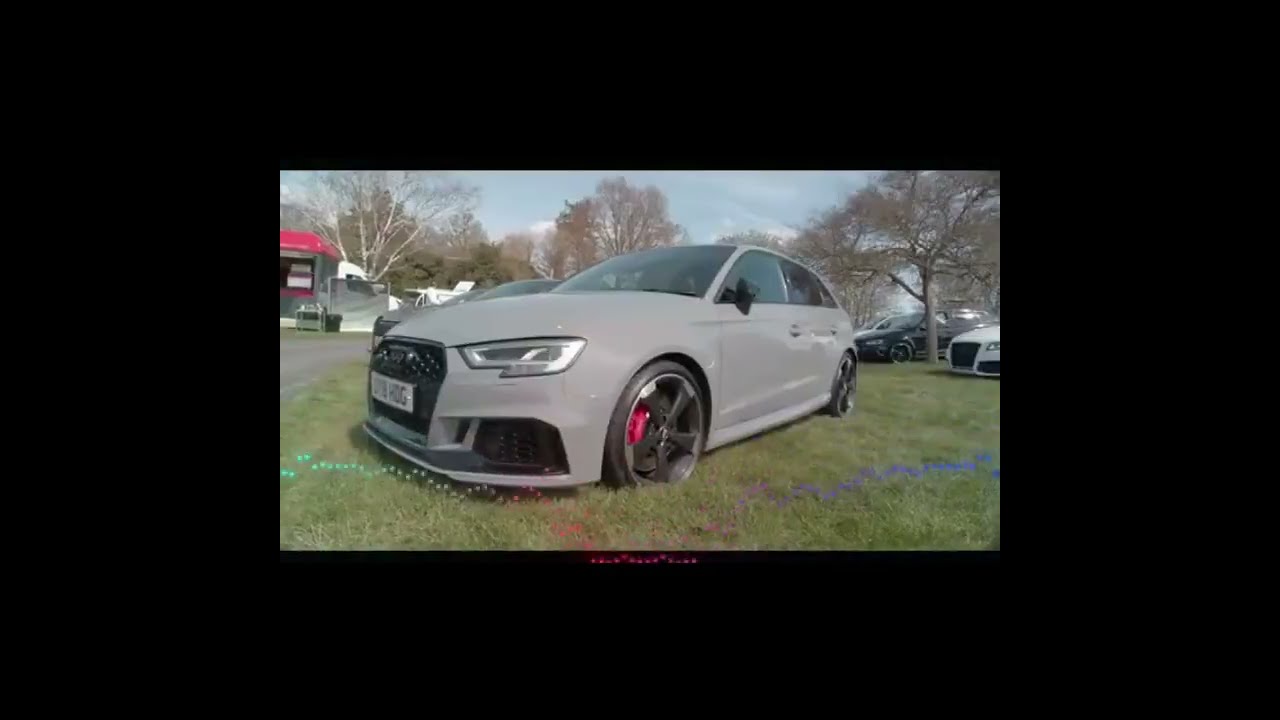This rectangular photograph is framed by a thick black matte border and features a color overlay. Taken from ground level, the image captures a sporty, low-line gray Ford hatchback four-door sports car from the driver's side at an angle. The car, which has European plates on the front and is parked on green grass, boasts distinctive five-spoked mag wheels and red brake calipers. It also features black-tinted windows and a black grille. To the front of the car, you can see a bit of the front license plate.

In the background, the sky is blue with occasional white clouds. The scene includes several leafless trees suggesting an early winter or early spring time of year. Additional cars, one white and one black, are parked further back, and a building, likely a shopping center or restaurant, is visible to the left. This building appears to have dining areas with white plastic tables and chairs. To the far middle left, a driveway is noticeable. A graphic is overlaid at the very bottom of the photo.